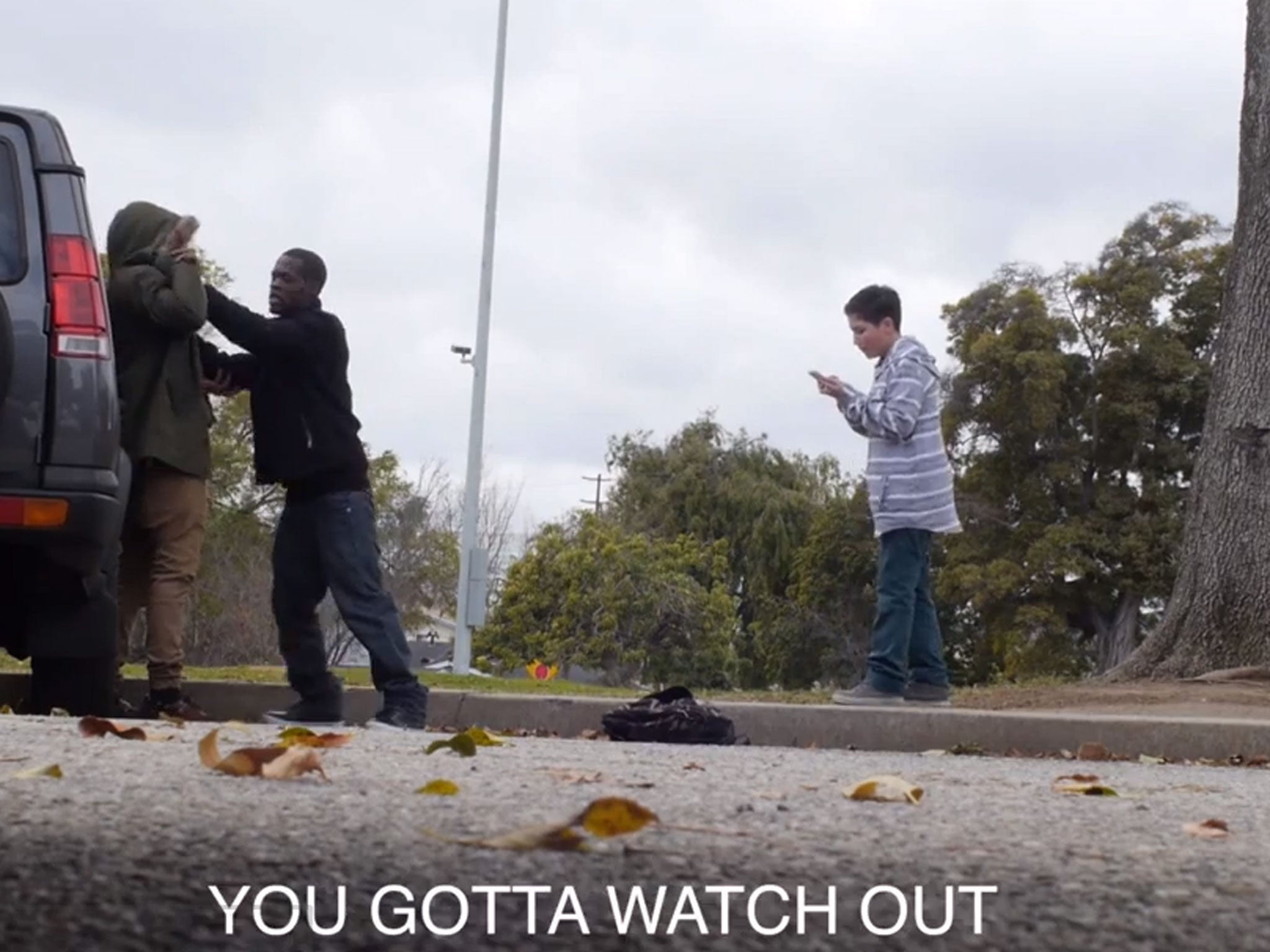The image depicts a tense confrontation in a suburban setting with a gray, cloudy sky above. Central to the scene, an African-American man wearing a black sweater, blue jeans, and black gym shoes is aggressively pushing another man against a gray truck. The man being pushed wears a green jacket with fur trim at the hood and beige pants. His back is pressed against the truck, which is parked facing away, positioned in the upper left corner of the image.

Behind the confrontation, a young child or possibly a small teenager is seen on a cell phone, seemingly indifferent to the struggle. This child, who has short black hair and a Caucasian appearance, is dressed in a gray shirt with white stripes and blue jeans. The background reveals a typical American suburban environment with buildings and green trees, along with a noticeable pole that could be a flagpole.

At the bottom of the photo, white text in all caps reads, "YOU GOTTA WATCH OUT," adding a sense of forewarning or urgency to the situation.